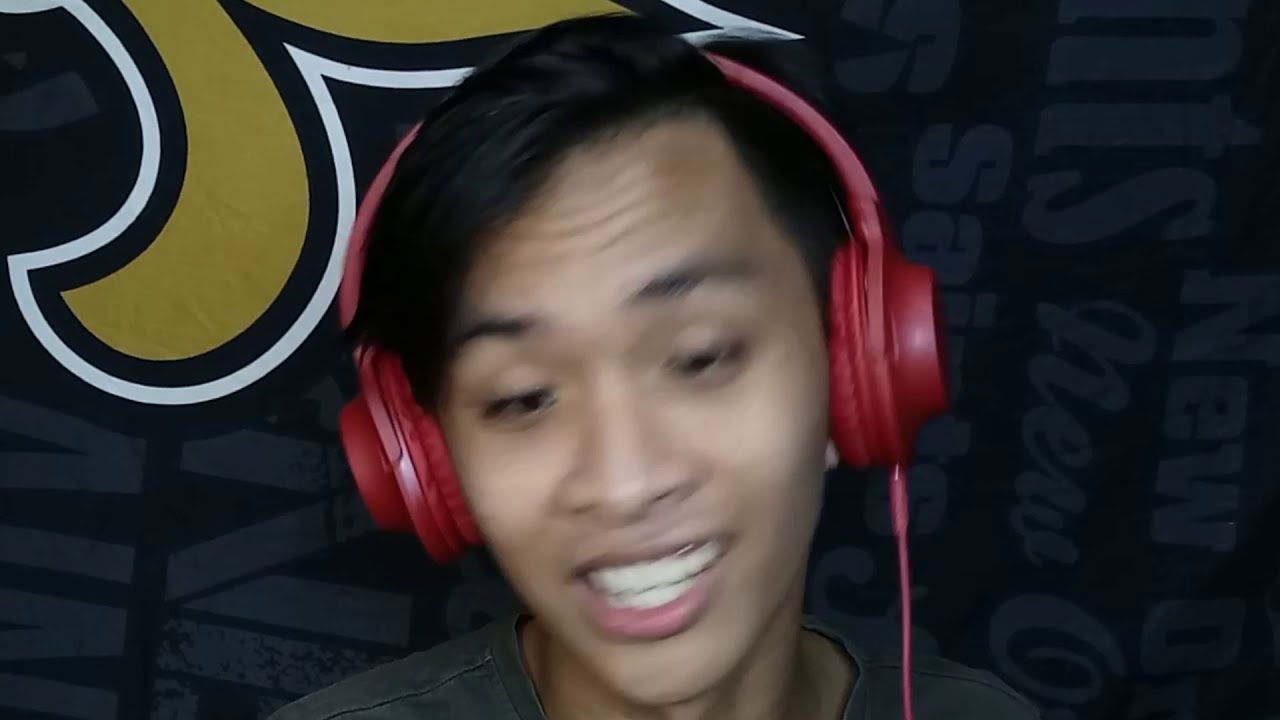A blurry photograph captures an individual of possibly Indian or Asian descent, wearing red headphones with a red cord dangling from his right ear. The man, who has short brown hair and medium-toned skin, is either smiling or speaking, displaying his white teeth. He is dressed in a dark, possibly gray, t-shirt. The background is somewhat obscured but appears to feature a navy blue tapestry or blanket adorned with vertically oriented dark gray writing. Additionally, there is an indistinct image resembling a mascot or logo in the top left corner, characterized by yellow curls outlined in black and white, reminiscent of the New Orleans Saints logo.